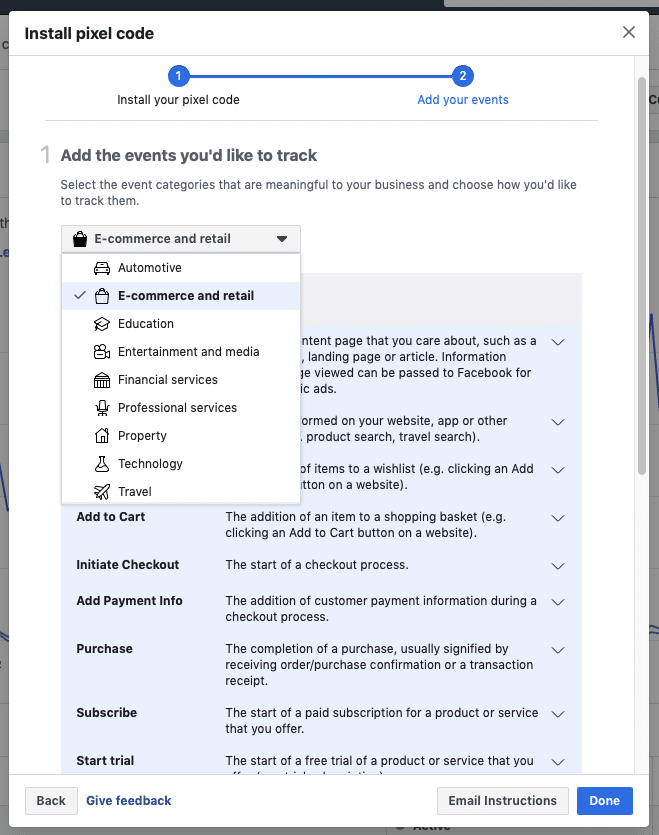A pop-up web page titled "Install Pixel Code" is displayed, marked by an 'X' button in the upper right corner for exiting. The upper left corner features the title in black text. Below the title, a blue progress bar spans the width of the pop-up, symbolizing the installation stages with '1' on the left indicating "Install Your Pixel Code," and '2' on the right, which the progress bar is aligned with, representing "Add Your Events."

The main body of the pop-up begins with a numbered step '1', instructing users to "Add the events you'd like to track." It elaborates with a guideline: "Select the event categories that are meaningful to your business and choose how you'd like to track them." Beneath this instruction exists an expanded drop-down menu titled "E-commerce and Retail," displaying "Automotive" as the first entry and "E-commerce and Retail" as the second. The latter is accompanied by a checkmark, indicating that "E-commerce and Retail" is the selected category.

Further down are multiple drop-down menus related to specific event actions, each with titles such as "Add to Cart," "Initiate Checkout," "Add Payment Info," and "Purchase." In the lower right corner of the pop-up, a small blue rectangular button labeled "Done" is visible, offering an option to finalize the steps.